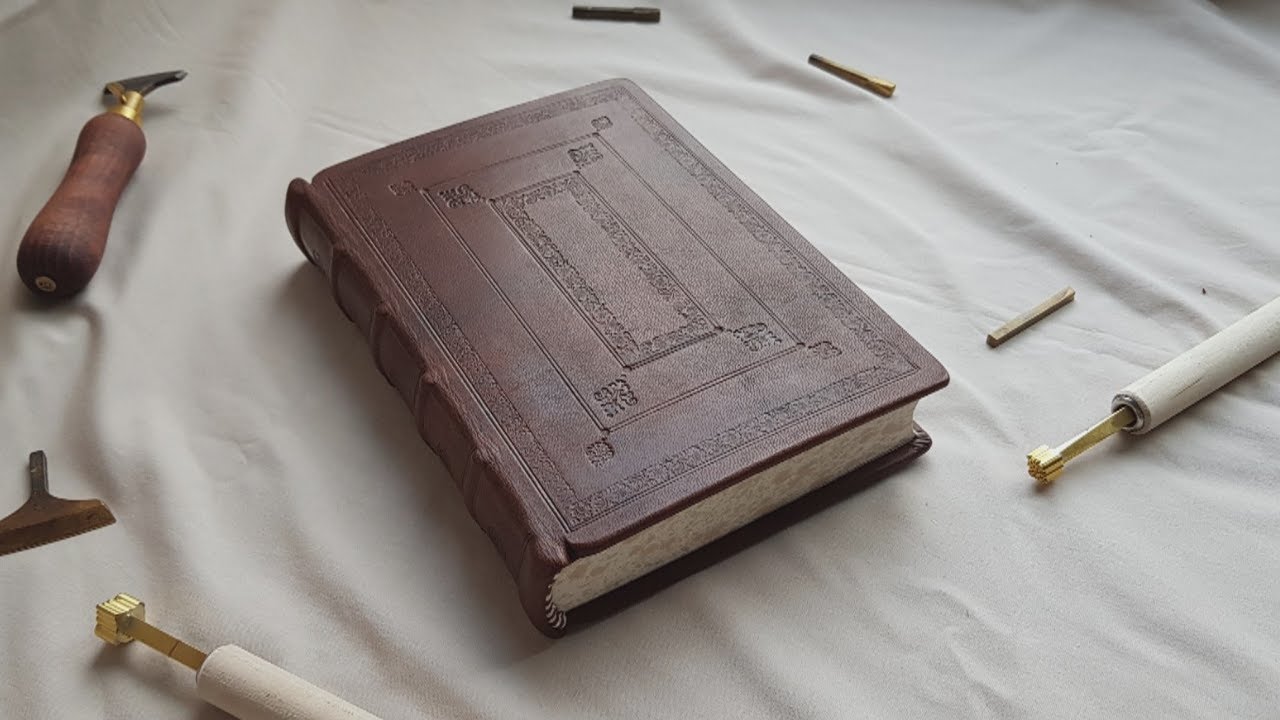In this photograph, a handcrafted brown leather hardcover book lies prominently in the center, resting on a slightly crinkled white fabric. The book’s cover features intricate embossing, including geometric and floral patterns, bordered by ornate engravings. Asian kanji characters are positioned within an inverted diamond shape on the cover, highlighting the detailed, delicate craftsmanship. The spine of the book has raised ridges that run vertically, adding to its tactile appeal. Surrounding the book are various chiseling tools, likely used to create the detailed patterns on the leather, reinforcing the artisan’s handiwork. The overall composition suggests a work-in-progress scene, capturing both the tools and the finely crafted book against the textured fabric background.